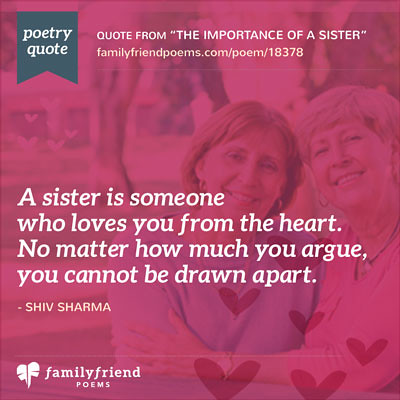This is a square poster with a red-pink overlay featuring an image of two older women on the right side, one with whitish-gray hair and the other with brownish hair, who appear to be smiling and hugging. In the bottom left corner, a small leaf symbol accompanies the text "Family Friend Poems." The upper left and upper right corners display ribbon icon banners with white text that read "Poetry Quote." Centered at the top, white text states: "Quote from 'The Importance of a Sister,' FamilyFriendPoems.com/poem/18378." Below this, there is a block of white text with the poem: "A sister is someone who loves you from the heart. No matter how much you argue, you cannot be drawn apart." The quote is attributed to Shiv Sharma.